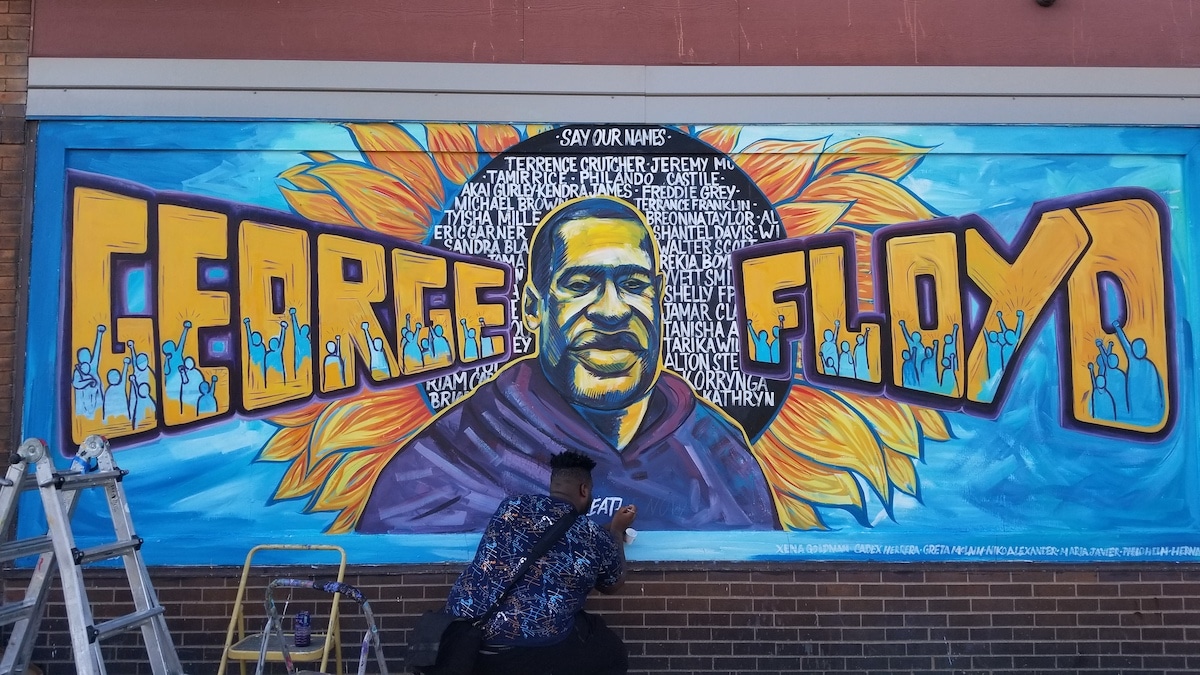The photograph captures a detailed and vibrant mural honoring George Floyd, set against a red brick wall. A person, identifiable as a Black man with short dark hair and wearing a bluish shirt, is seen kneeling on a small stepladder, painting the mural from behind. The mural is a large rectangle with a predominantly black background. 

In the center of the mural is a striking image of George Floyd, depicted with a short-trimmed beard and hair, and wearing a dark hoodie, looking directly at the viewer. His skin is rendered in a yellowish tone, accentuating his broad nose and large lips. Surrounding his head is a black circle with white lettering that reads "Say Our Names." Radiating from this black core are yellow and orange leaves with a blue outline, evoking the aesthetic of a sunflower.

To the left of Floyd's portrait, the word "George" is painted in a yellowish font, and to the right, "Floyd" is similarly displayed. At the base of each letter, blue silhouettes of people with raised fists can be seen, symbolizing solidarity and protest. Within the black circle, several names such as Terrence Crutcher, Jeremy Moo, Tamir Rice, and Philando Castile are visible, though some are obscured by Floyd's image, each representing a life lost to systemic injustice. This poignant artwork blends elements of remembrance and resistance in a visually powerful tribute.